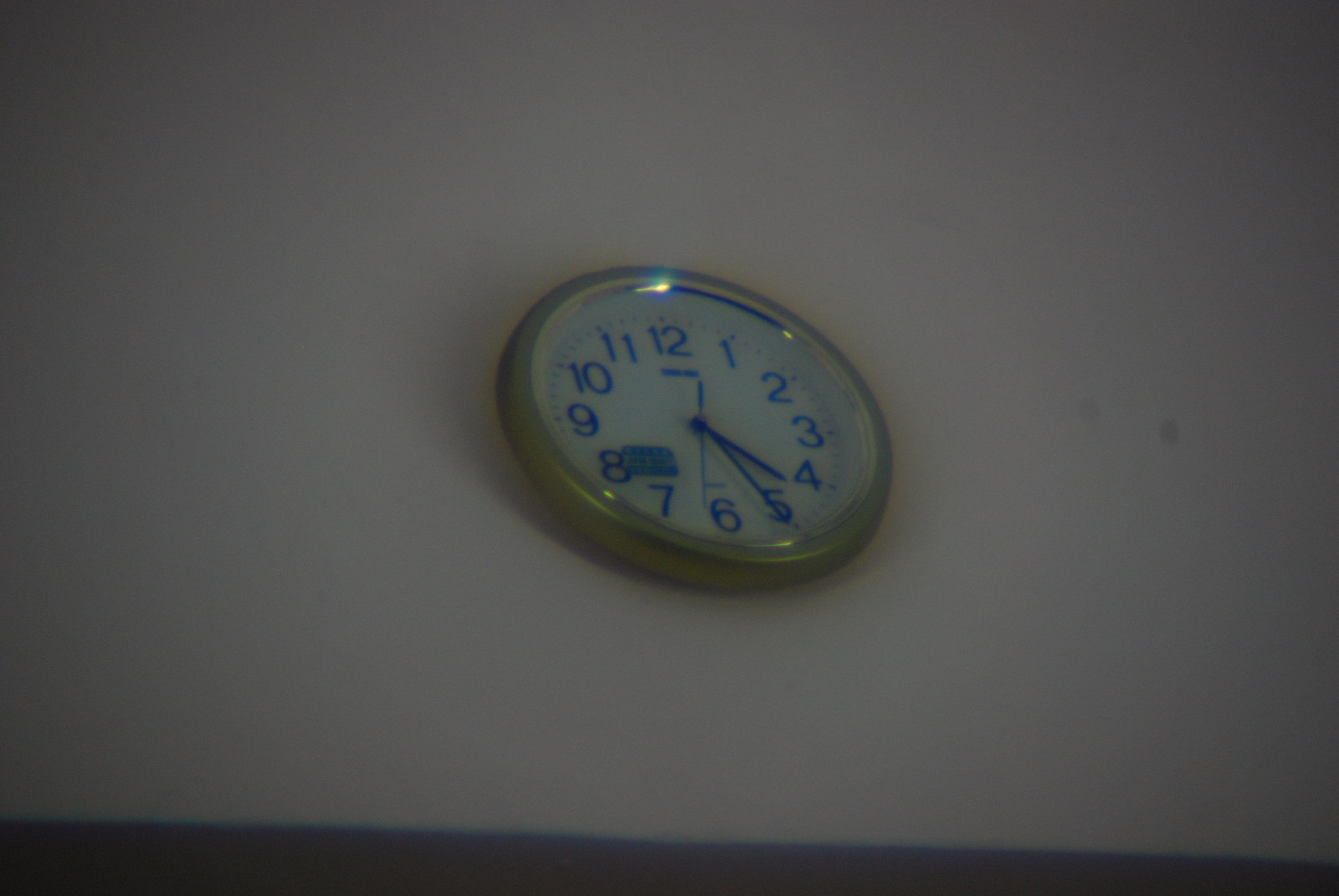The image features a silver or gray metallic clock with a highly reflective surface, mounted on a white wall that mirrors its sheen. The body of the clock is round and made of a durable, polished metal that catches the light. At the top left and right corners of the image, there are blocks—specific details about these blocks are not provided, but they frame the clock. The bottom portion of the image is shaded, accentuating the bright reflective top part of the clock.

The clock face is classic, with numbers ranging from 1 to 12. The hour hand points to the 4, the minute hand is at the 5, and the second hand is positioned between the 6 and 7. The clock hands are designed in a cohesive style, with all three connected at the center pivot. There appears to be text at both the top, likely indicating a brand name, and the bottom of the clock face, although the exact content of the text is not discernible.